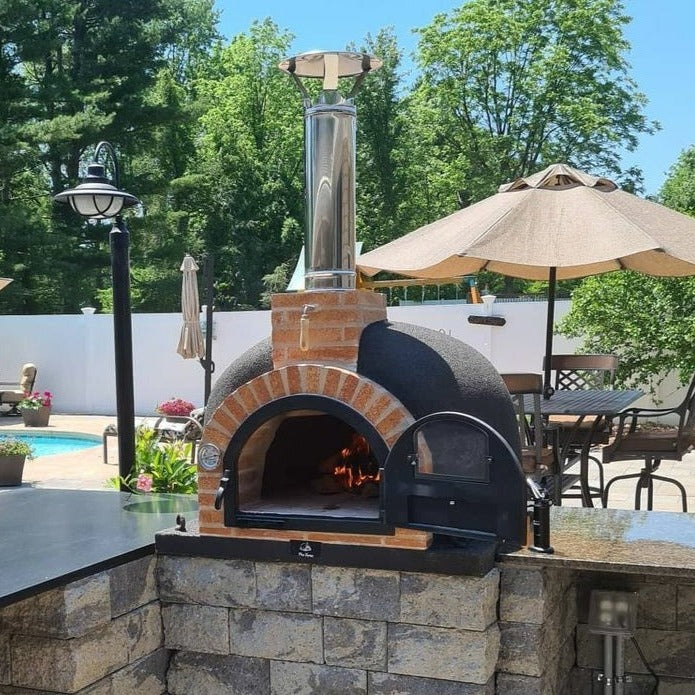This image captures a picturesque outdoor scene in a backyard, showcasing a central, semi-circular red brick and black stone pizza oven. The oven is set on a gray brick paver wall, topped with a sleek granite countertop, and features an open door revealing a fire burning inside. A shiny stainless steel chimney extends upwards from the oven. To the right of the oven, there is a black and brown countertop which potentially includes a unique black torch or lamp. The oven area is complemented by additional plug-in outlets underneath the countertop.

In the left background, a clear, inviting swimming pool is visible, accompanied by large planters filled with vibrant flowers and plants. To the right, a table and chair set with an open brown umbrella sits on the patio. A stylish white fence lines the yard, marking the property's boundary. Beyond the fence, lush green trees sway gently under a bright blue sky, indicating a warm spring or summer day.